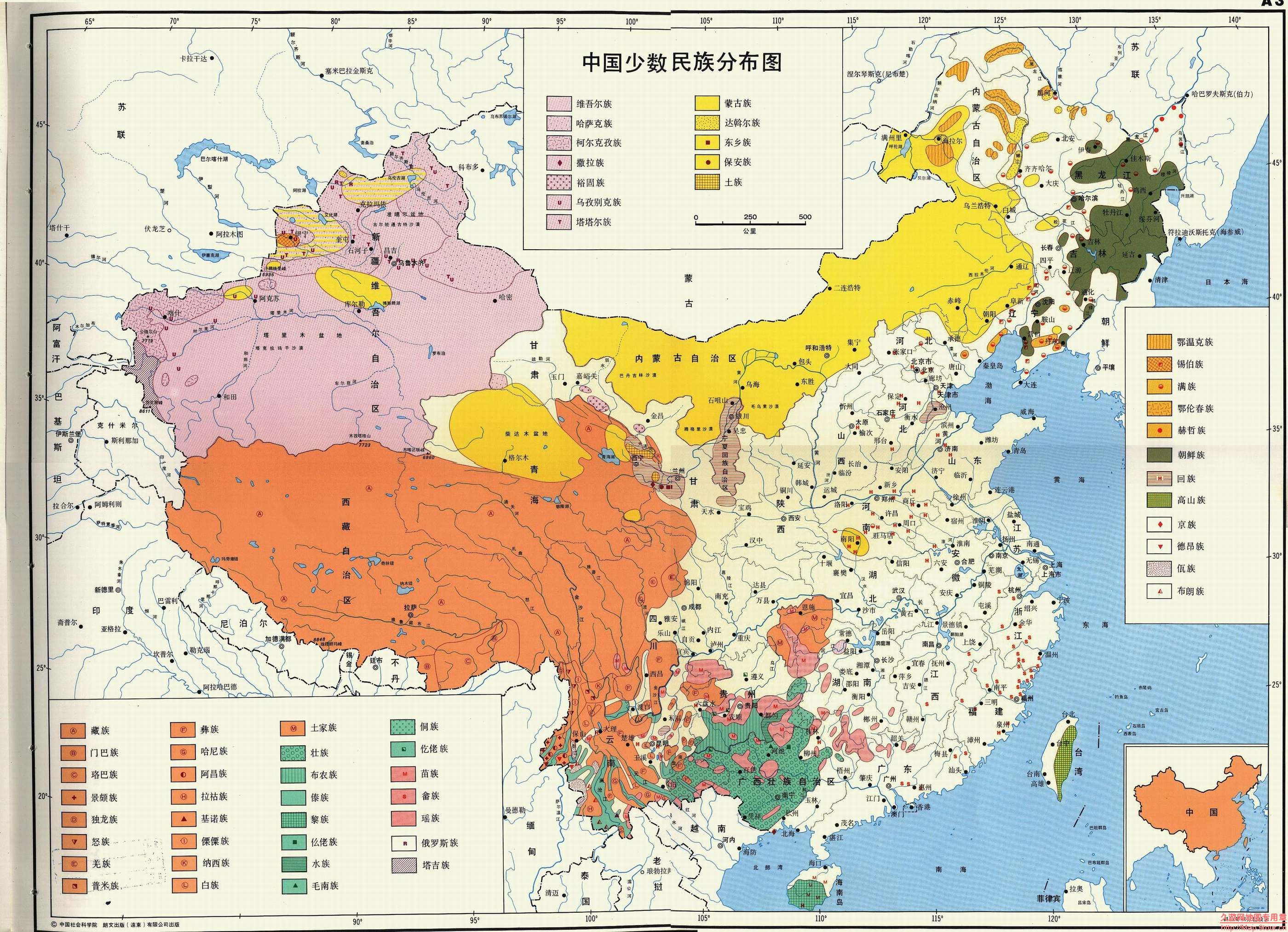This image features a detailed map of what seems to be Asia, predominantly white, with a complex array of coded regions in vibrant colors. The text is in an Asian language, possibly Japanese or Mandarin. The colored regions include a light purple country, a yellow country, an orange-red country, and both light and dark green countries. A prominent blue area occupies much of the lower to upper right side, suggesting a significant body of water and two islands. At the top center, there's a small box containing writings, with a set of purple blocks to the left and yellow blocks to the right. The map includes a series of labels and codes, though their meanings are not known. On the lower left, there is another notable box displaying rows of red, green, blue, and white blocks, each presumably corresponding to specific areas on the map. Individual regions and landmarks are marked with various colors, offering a visually rich representation of geographical and possibly political divisions.